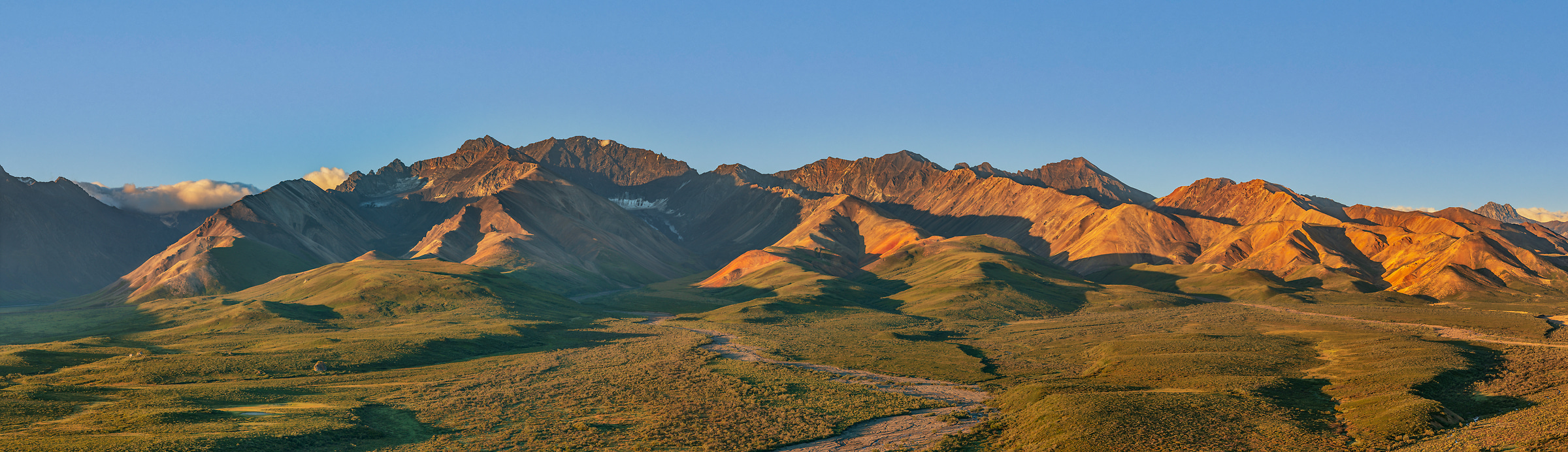This panoramic image captures a sweeping view of a remote mountainous desert range under a clear blue sky, likely photographed during the golden hours of sunrise or sunset. The vast mountain range stretches horizontally from the left to the right side of the image, with ridges glowing in vibrant hues of orange-red, suggesting the warmth of the sun. The left side of the mountain shows small patches of snow nestled in its crevices, and delicate, golden-tinted clouds hover above. 

In the foreground, verdant grasslands and meadows are visible, along with dry riverbeds and footpaths leading towards the mountains. The sky is mainly clear, revealing only some marine layers of fog resting atop the peaks, contributing to the tranquil, expansive atmosphere. The image's wide-angle or possibly stitched format accentuates the remote, untouched beauty of this majestic landscape, free from any man-made structures or roads.